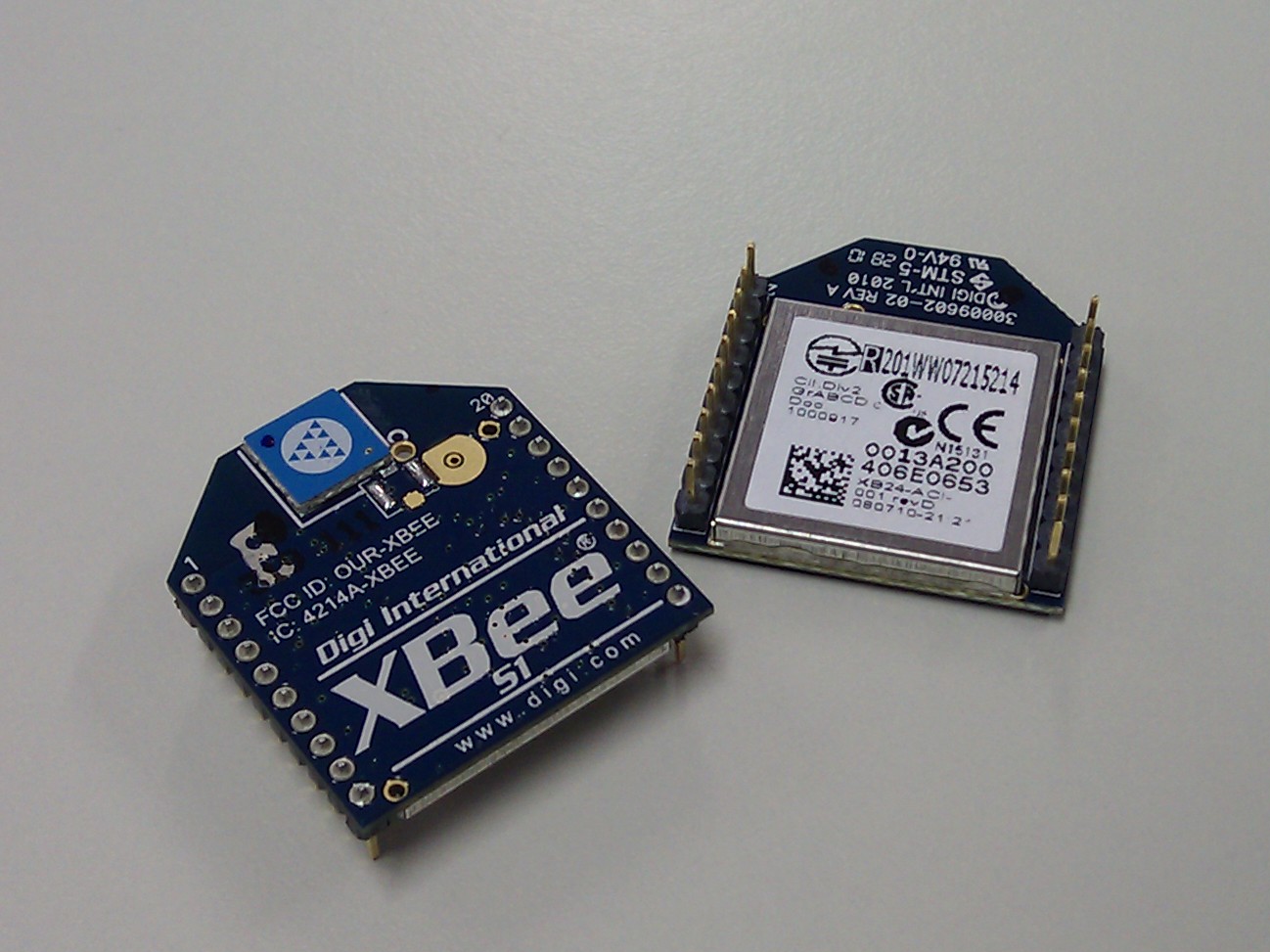The photo depicts two navy blue microchips against a gray background, both branded as Digi International XBEE. The chip on the left, positioned upright, reveals detailed branding and technical information. It prominently displays the Digi International logo, followed by large text that reads "XBEE S1." Above the logo, smaller text includes "FCC ID: OUR-XBEE" and "IC: 4214A-XBEE," with the company's website "www.digi.com" printed at the bottom. This chip also features a design with a yellow circle, a blue square, a white circle, and blue triangular shapes. The other chip on the right is flipped upside down, showing the base and the serial number. Both chips have different size lettering and are angled opposite each other – one to the right and the other to the left.